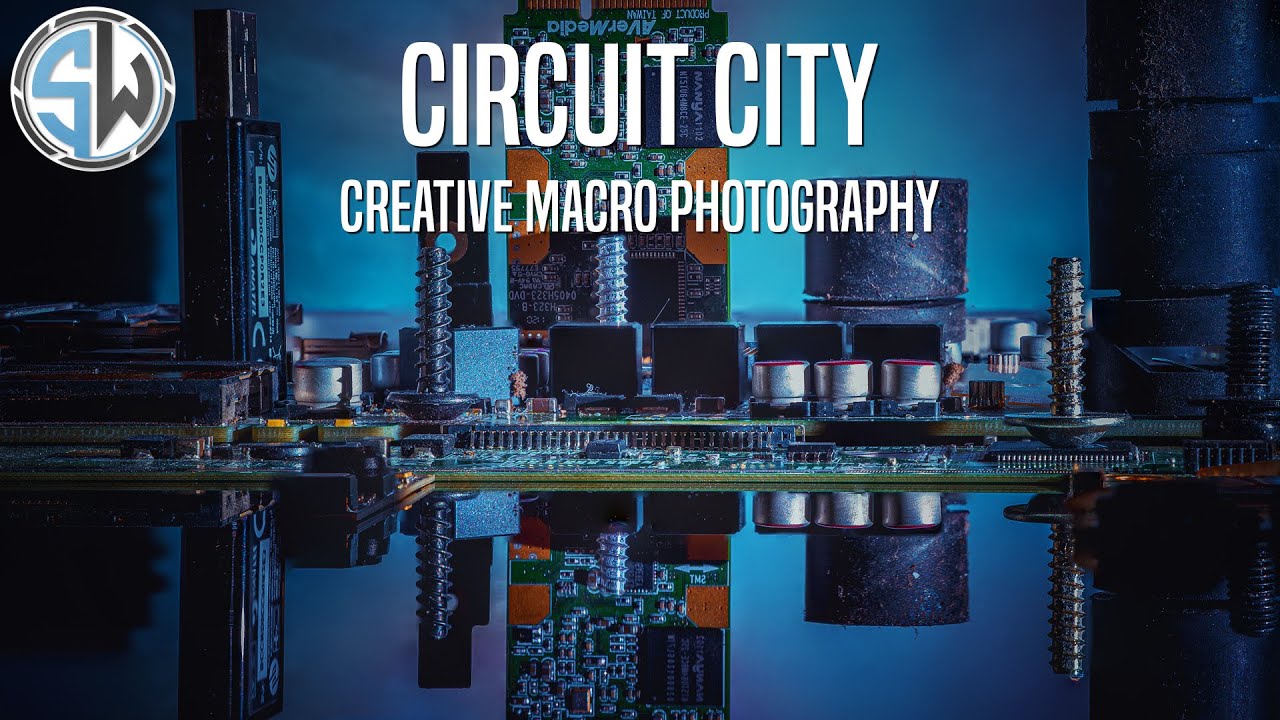This advertisement features Circuit City Creative Macro Photography, showcasing a meticulously detailed image of a circuit board, possibly from a PC motherboard. The focal image, tinted in a cool bluish hue, highlights various computer components such as chips, screws, and other intricate parts. Notably, the photograph employs a mirrored effect, doubling the intricate visuals and enhancing the depth of the composition. In the upper left corner, a logo appears within a white circular background, enclosing a stylized blue "S" and a gray "W" surrounded by a gray ring. The text "Circuit City Creative Macro Photography" is prominently displayed in white at the top, reinforcing the ad's purpose and brand identity.